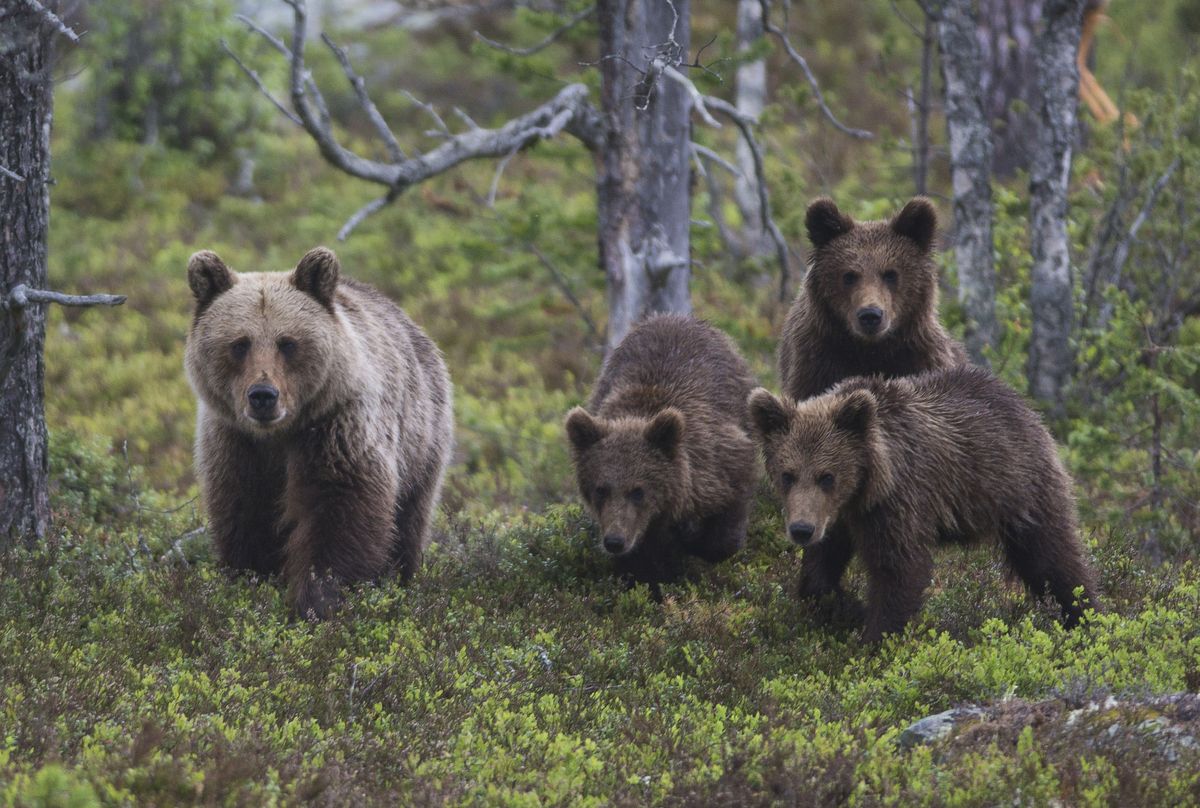This detailed photograph features a family of bears in a sparse forest setting with thin, pale-barked trees and a ground covered in low-lying greenery and moss. In the foreground stands a large adult bear with a thick, shaggy coat that is a grizzled blend of light and dark brown. Its eyes are focused and its ears are perked as it gazes directly at the person taking the picture. Positioned to the right, three younger bears—clearly cubs—display fur that is more uniformly brown, soft, and fluffy. The cubs are arranged in a triangle formation, with two at the base and one on top, all exuding a curious, innocent look. The smallest cub on the far right appears particularly attentive, with ears pointed straight up. All four bears are alert and wary, staring intently at the camera, creating an atmosphere of cautious curiosity. The overall scene is tranquil yet captivating, capturing a rare, intimate moment in what seems to be a Canadian forest.